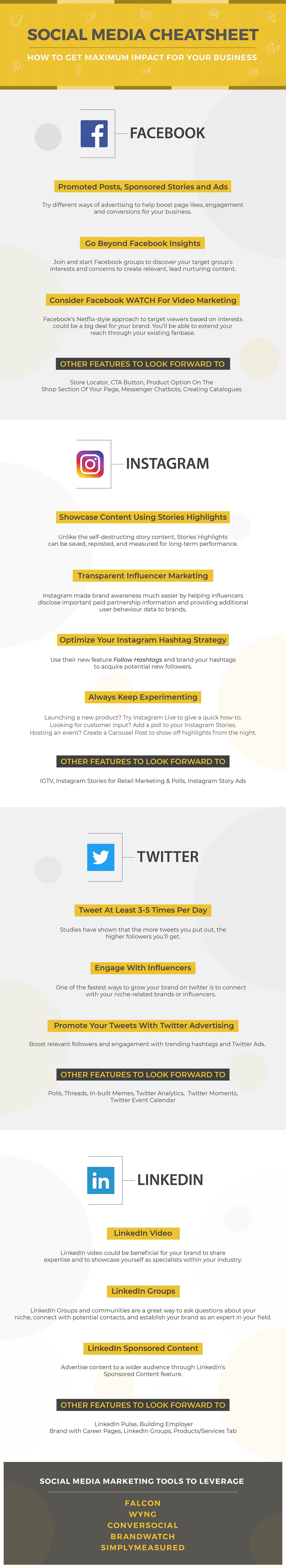The image is a detailed yet cluttered "Social Media Cheat Sheet" designed to help businesses maximize their impact on various social media platforms. The page features large, somewhat legible headers for Facebook, Instagram, Twitter, and LinkedIn, but the smaller text is nearly unreadable due to the crammed layout and poor contrast. There are several links at the bottom with slightly better readability against the background, promoting social marketing tools such as Falcon. The background of the image varies between white and light gray, with predominantly black text. Despite its intended purpose, the readability issues make it difficult to extract specific actionable information.